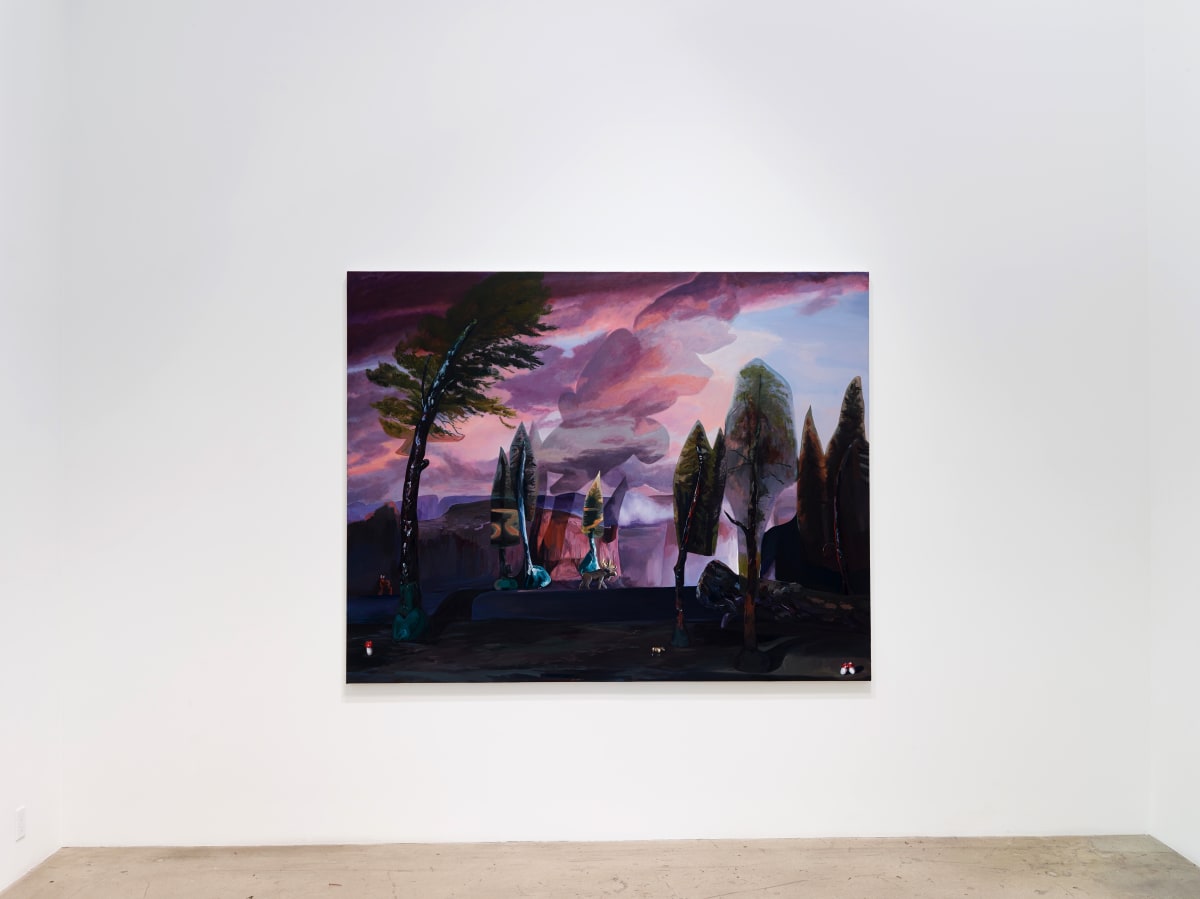In an art gallery with pristine white walls and a polished brown floor, hangs a solitary painting, drawing immediate attention with its intriguing details. This rectangular artwork, roughly six inches wide by four to five inches high, appears to be created with watercolors or possibly oils, favoring a cartoon-like style over realism. The scene depicted shows trees swaying under the influence of a strong wind, their branches leaning to the right. The sky above is an expressive mix of pink and purple clouds, giving a sense of dynamic movement from left to right, culminating in a serene blue patch in the upper right corner.

At the painting’s center, an assortment of rock formations or steps ascends toward what appears to be an entrance to a castle-like structure. Purple-toned buildings rise above this platform, adding to the surreal, whimsical atmosphere. To the right, a tree's branches are outlined, almost as if encased in a plastic covering, while a tall pine tree stands in contrast on the left, its lower branches missing.

Throughout the composition, the trees and plants exhibit a geometric intricacy, with leaves and branches painted in angular, abrupt turns. The floor and a small portion of a wooden table with inverted sides are visible at the bottom of the photograph, grounding the ethereal scene in a tangible reality. The overall color palette, dominated by purples, pinks, and blues, enriches the enchanting aura of this solitary, thought-provoking piece.